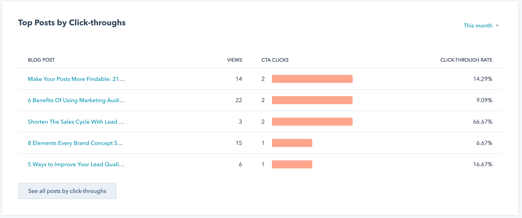A small horizontal rectangular screenshot titled "Top Posts by Clickthroughs" occupies the upper portion, featuring several columns of information. The first column, labeled "Blog Post," lists five entries in blue text. Adjacent to it, the second column displays "Views" for each blog post. Directly next to the views, a third column illustrates the "Clicks" received by each post, augmented with a bar graph for a visual representation comparing click numbers. The far-right column is labeled "Clickthrough," showing the clickthrough rates as numerical percentages for each corresponding blog post.